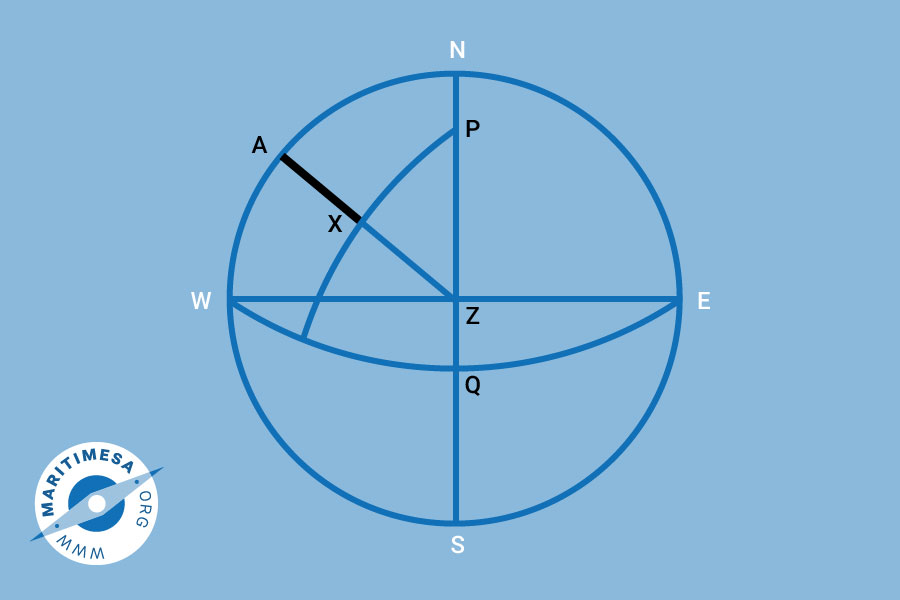The image is a detailed diagram set against a pale baby blue background. Central to the graphic is a blue circle that resembles a compass or a globe. This circle is divided into four quadrants by a vertical and a horizontal blue line, each labeled with compass points: N (North) at the top, S (South) at the bottom, W (West) on the left, and E (East) on the right.

Notably, several additional lines and letters are marked within the diagram. A line labeled P runs vertically from N to S. Horizontally across the center, there’s a line marked Z, running from W to E. Between N and W, another line labeled A intersects the quadrant, with an X positioned along this line. Also prominent is a curved line labeled Q in the lower section, suggesting a pathway or an axis.

In the upper left quadrant, multiple crisscrossing lines add complexity to the diagram, including a notable arc. Outside the circle, in the bottom left corner of the image, a white circle contains a smaller graphic resembling a protractor, alongside the text “Meritamesa.org” and the website “www.meritamesa.org.”

Overall, the image serves as a complex navigational or directional illustration, possibly related to compass bearings or geographic positioning.